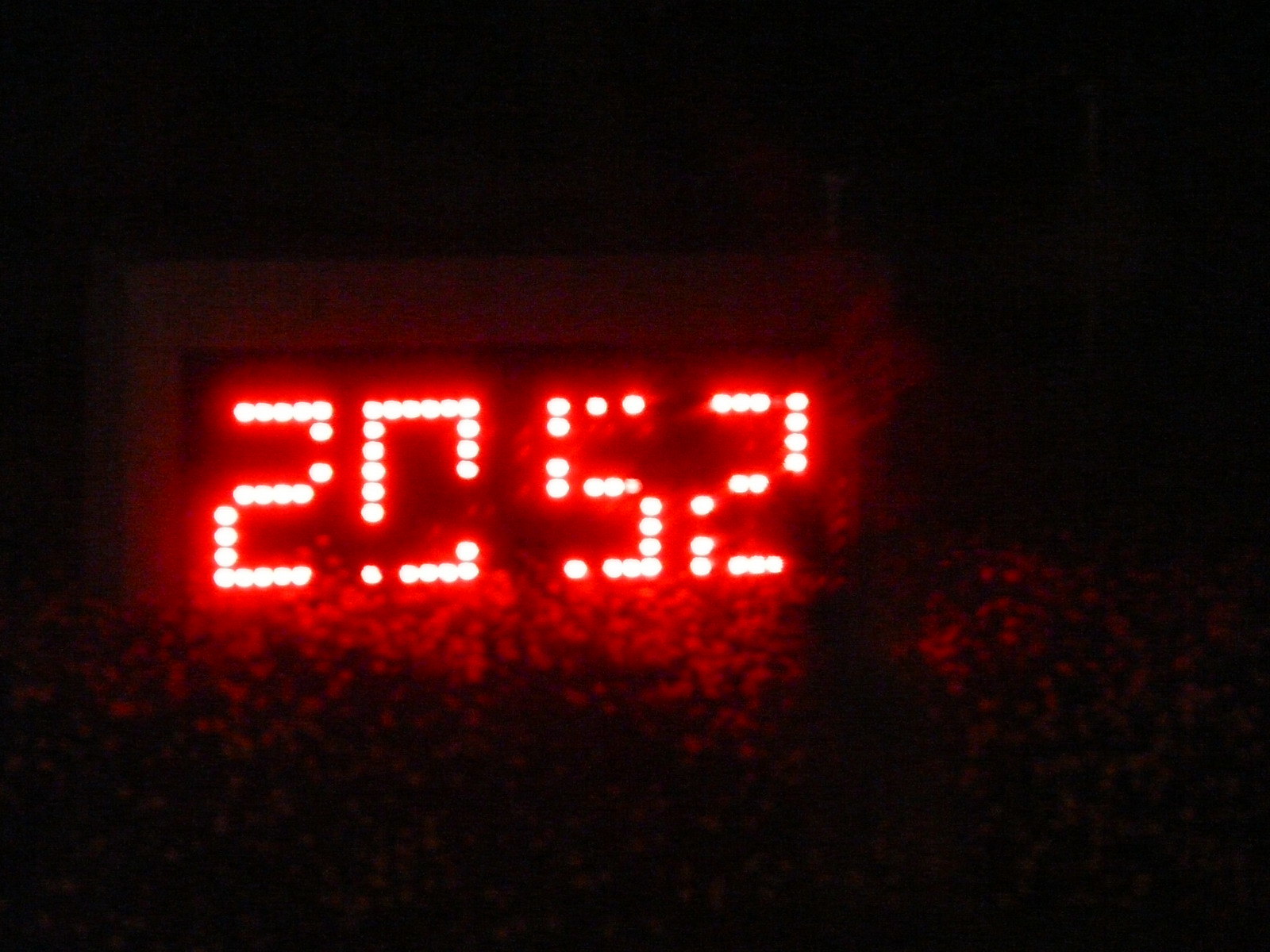In a dimly lit scene, a large digital clock dominates the focal point with its striking red numerals that display the time "20:52." The digits, illuminated by an array of small white diodes, emit a vivid red glow. Encircling the clock face is a barely discernible gray-colored border, shrouded by the surrounding darkness. The clock appears to be situated outdoors, suggested by foreground foliage and a hedge that nearly reaches the base of the glowing numbers, adding an air of mystery to the overall setting.